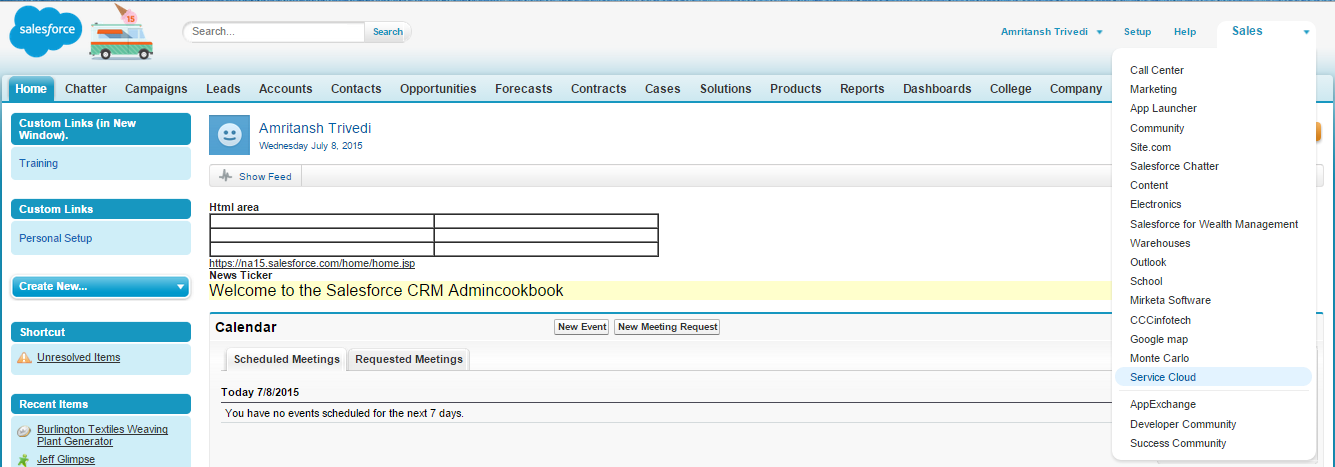At first glance, this appears to be a website interface, zoomed in at 150% for detailed viewing. The top of the page features a graphic element, possibly a truck adorned with an American flag, along with a search box. On the upper right corner, there are several labels, although some text is not entirely readable. Identifiable labels include "Setup," "Help," and "Sales," with the "Sales" drop-down menu currently expanded. This menu contains approximately 20 items, one of which, "Service Cloud," is highlighted.

Moving to the main area of the website, a series of tabs are visible across the top. These tabs include: Home, Chatter, Campaigns, Leads, Accounts, Contacts, Opportunities, Forecasts, Contracts, Cases, Solutions, Products, Reports, Dashboards, and Company, although the full list is partially obscured by the open sales menu.

On the left-hand side, there's an additional column with smaller items and custom links. The main content section of the page prominently features the heading "Armished," which could be a user's name, indicated by an accompanying smiley face profile icon. Below this, there is an empty text box segmented into six lines, followed by text that reads, "Welcome to the Sales First CRM Admin Cookbook." Additionally, a calendar is displayed, featuring scheduled meeting times and related information.